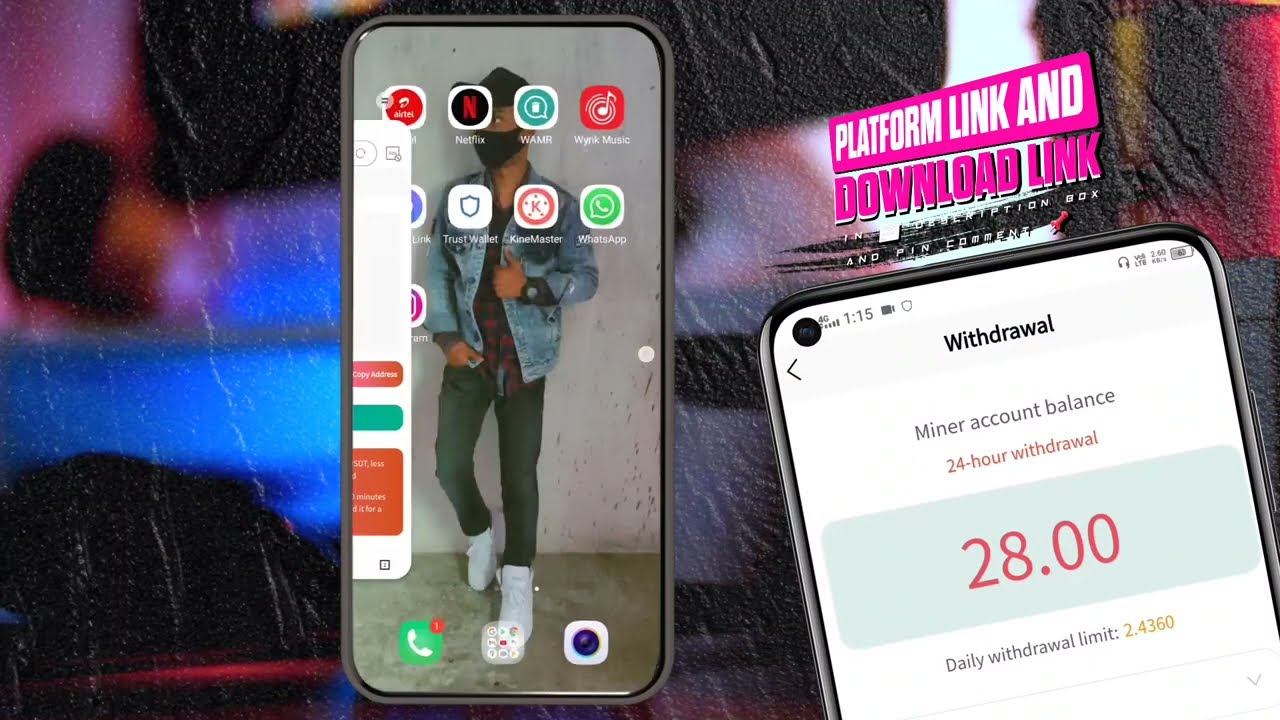The image is an advertisement for a mobile app, featuring a dual layout with two prominent cell phone screens against a blurred, colorful background. The left side of the graphic showcases a phone mock-up with a home screen displaying various apps overlaid on an image of a brown-skinned man in a black ball cap, black surgical mask, denim jacket over a red flannel shirt, black jeans, and white sneakers. Visible apps include Netflix and some music apps, with a green phone icon indicating one call at the bottom. To the right, there's a close-up of another phone, partly cropped and tilted left, displaying a banking app. The screen shows text such as "Withdraw," "Minor Account Balance," and "24-Hour Withdrawal: $28" in red, with a daily withdrawal limit of "24360." Above this phone is a pink banner with white text saying "Platform Link and Download Link," accompanied by a thumbtack emoji. The backdrop of the advertisement is a blurred scene with shades of blue, black, red, and pink, resembling rain on a window.